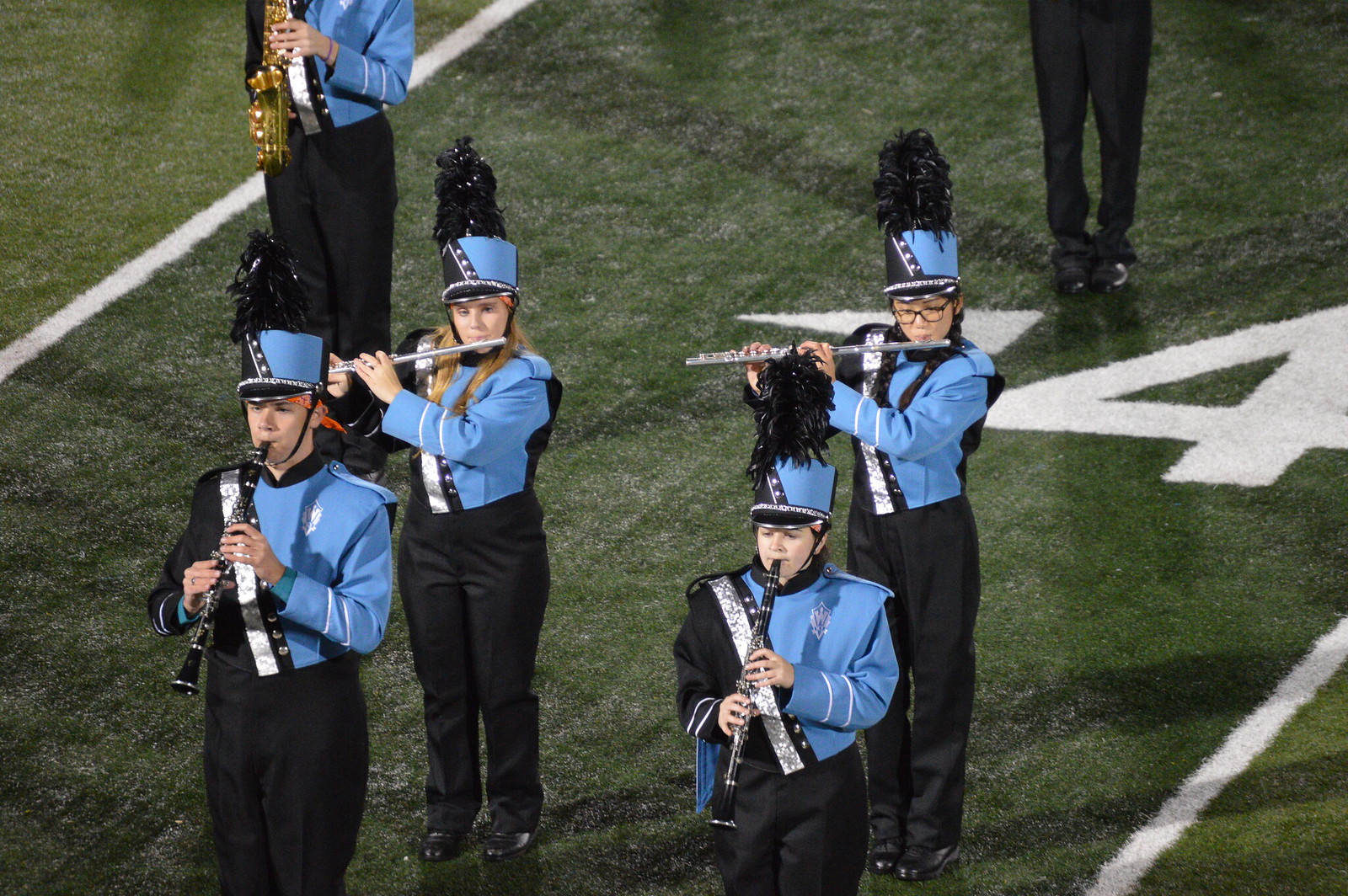This photograph captures a top view of a marching band on a green football field marked with white lines and a large number four. Centrally, four musicians are arranged in a square formation. Each musician is dressed in a blue jacket with silvery stripes, black pants, and a blue hat adorned with a large plumed black feather. In the front row, two musicians are playing piccolos, though initially misidentified as clarinets. Directly behind them, two other musicians are playing flutes. On the left, partially visible, is a fifth musician seen from the shoulders down, playing what appears to be a saxophone. Additionally, just the legs and shoes of a sixth musician can be seen on the right, leaving their instrument unidentified. This detailed assembly evokes the disciplined and coordinated spirit of a marching band performing on a prominent football field.